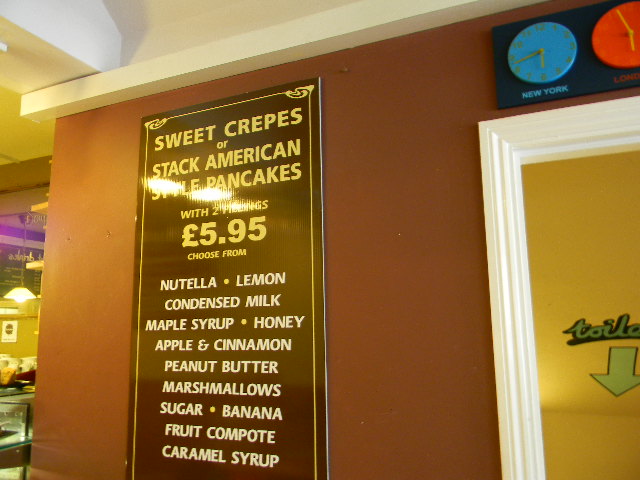This is a horizontal color photograph of a restaurant's menu displayed prominently on a wall. The menu prominently features a selection of sweet crepes and American-style pancakes, priced at £5.95. Patrons can choose from a variety of toppings, including Nutella, lemon, condensed milk, maple syrup, honey, apple and cinnamon, peanut butter, marshmallows, sugar, banana, fruit compote, and caramel syrup. Positioned above a doorway labeled "Toilets," two clocks are mounted on the wall, one labeled "New York" and the other "London." The image captures a glimpse of the restaurant's ambiance, with visible lights, additional menus, and display cases around the corner. The warm lighting enhances the inviting atmosphere of the space.